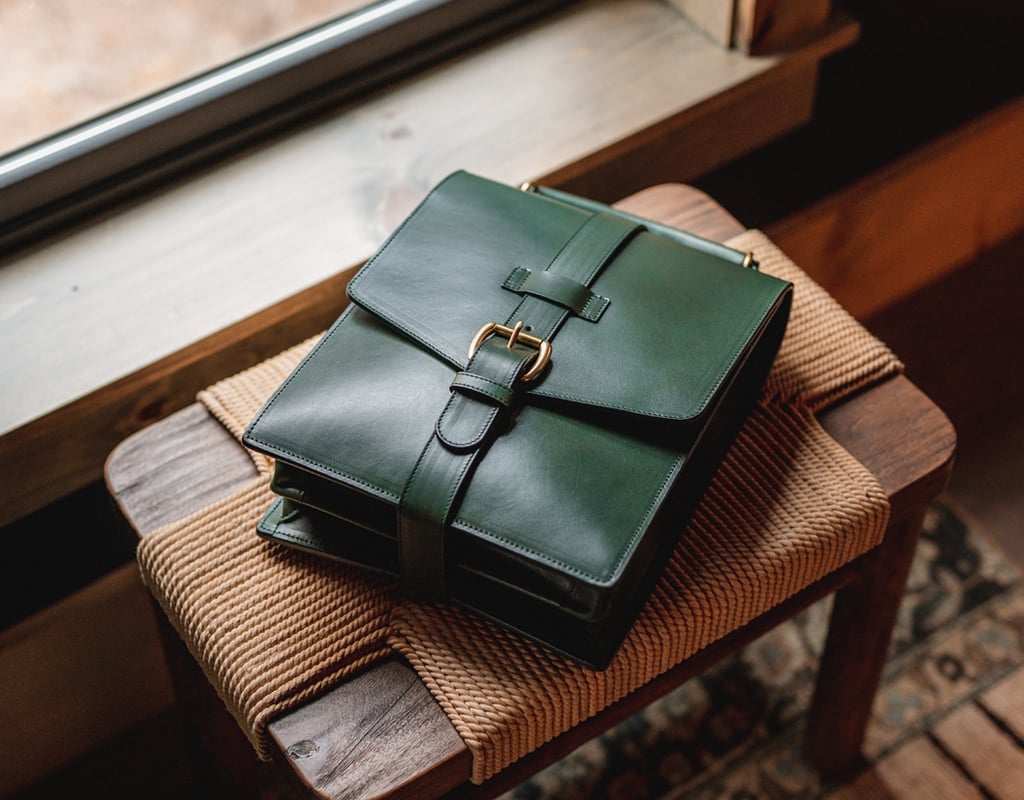The high-definition photo captures a dark green leather saddle bag with intricate stitching. The bag, which is square and of substantial size, has a distinctive belt-like strap that fastens over its front with gold buckles. It rests on its back, taking up about three-fourths of the surface area of a wooden stool. The stool itself features a cord-braided brown tabletop with a cross-shaped rope pattern. The setting includes a blurred background that reveals a wooden windowsill with part of a window visible in the upper left corner. The stool stands on a patterned tan area rug embellished with green and brown designs, adding to the rustic ambiance of the scene.